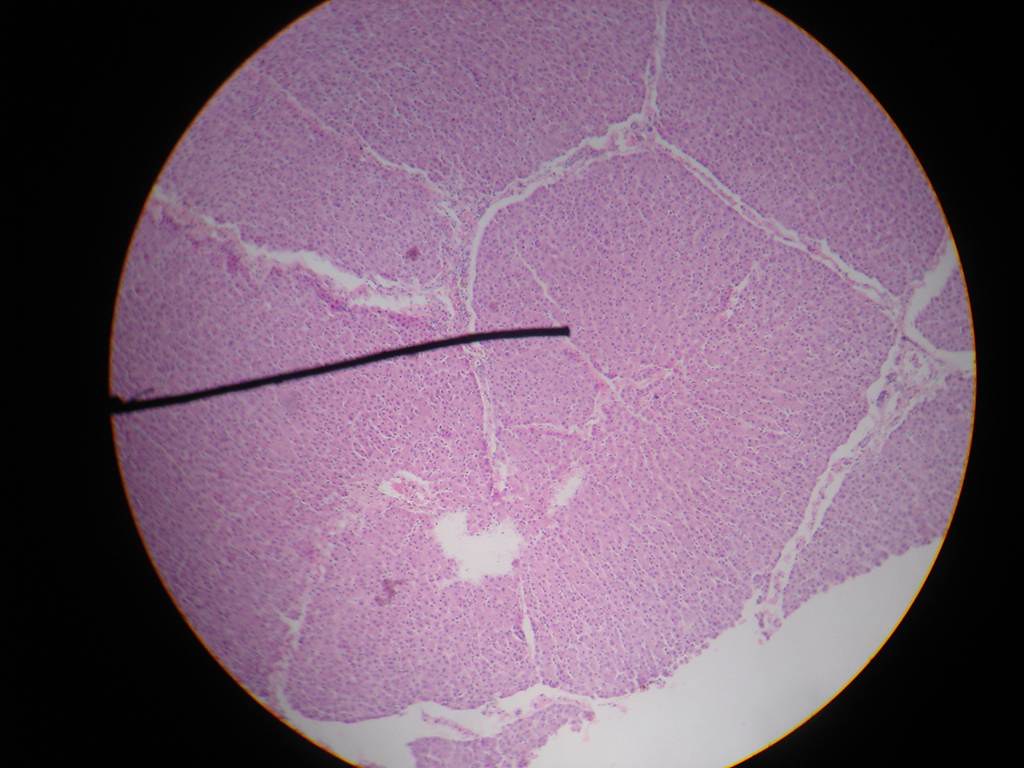This image appears to have been taken through a microscope, capturing a close-up view that resembles dried skin or a planetary surface. The focal point is a perfectly circular area dominated by a pinkish-purple hue, interspersed with intricate, white cracks that traverse the entire surface. As the image transitions toward the bottom, the color lightens, eventually becoming white, suggesting a thinner or less dense material in this region.

Adding to the complexity of the image, a significant black shadow, straw-shaped or hair-like, stretches diagonally from the left edge towards the center, partially obscuring the view. This shadow could indicate the presence of a contaminant, such as a hair or fiber, on the microscope slide. The texture within the circle is accentuated by tiny dots and web-like lines, contributing to the overall impression of a detailed, microscopic landscape. The background remains stark black, emphasizing the striking details within the circular frame.